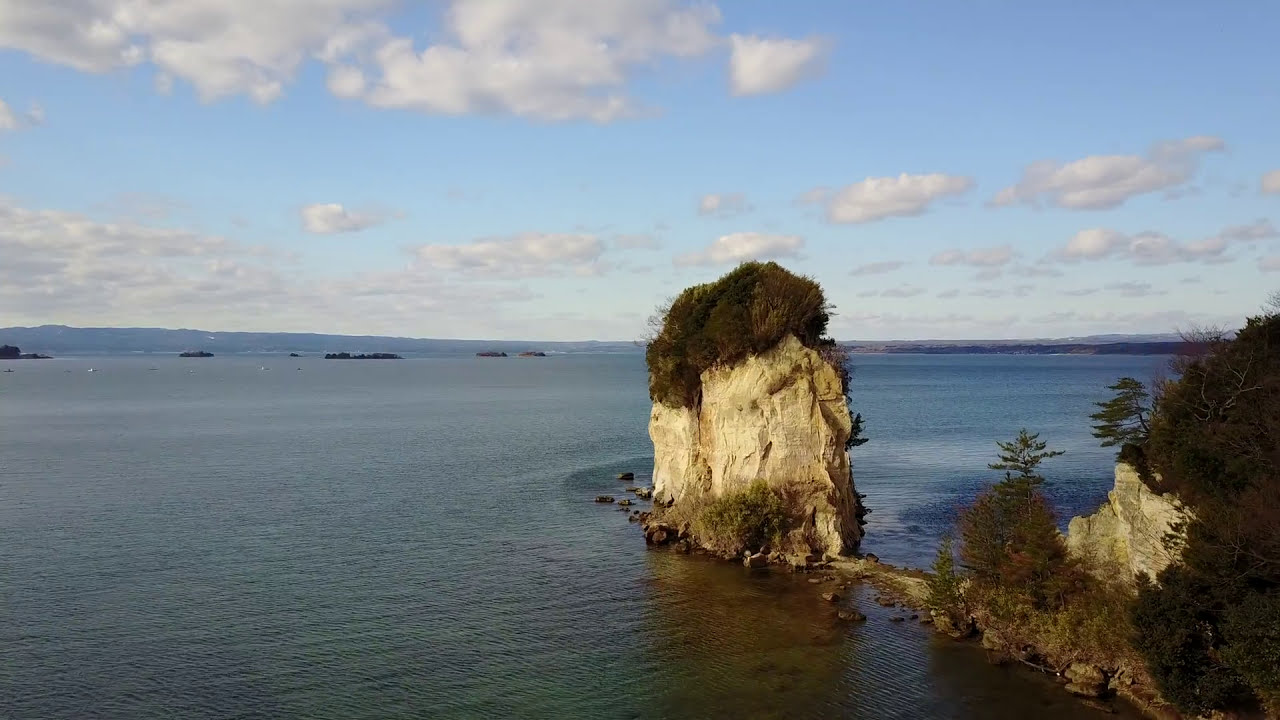In this picturesque scene, we observe a tranquil ocean setting punctuated by a massive, white boulder that juts dramatically from the water’s surface, extending upwards with verdant foliage, including bushes and trees, adorning its top. To the right of this boulder, we see an extension of land that resembles a hilly structure covered in the same green vegetation, suggesting the boulder was once part of this landmass but has since separated over centuries. The water surrounding the boulder is a deep greenish-blue, opaque and rich in color. In the distance, additional small rocky hills and dark shapes, possibly boats, can be faintly discerned against the horizon. This scene is framed by a vivid blue sky with scattered white clouds, bathed in sunlight, suggesting a clear daytime setting. Farther back, subtle hills emerge, completing the serene landscape.